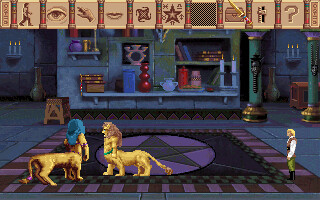In the center of the image, there is a notable grey star surrounded by several triangles positioned at the top, right, bottom, and left, creating a symmetrical pattern with a central shape. The surrounding area is predominantly blue, contrasting with patches of brown. To the right, there are distinct figures: green ants, blue boots, a brown tank, a person wearing a white shirt, and a blonde-haired individual. On the left side of the image, two lions are featured; the one on the left dons a blue hood and stands beside a humanoid figure with a yellow body. The background showcases shelves filled with various artifacts, including a red jar and a white jar. The pixelated nature of this video game image is further detailed by icons arranged at the top. There are six primary icons followed by a square and three additional icons. The top-left section includes a walking icon, an eye icon, and an X icon. These icons are separated by pillars, characterized by brown centers, blue tops, and red bottoms. Further icons include a hand icon, a lip icon, a star with surrounding symbols, a checkerboard, a chest with a sword, and a question mark icon.